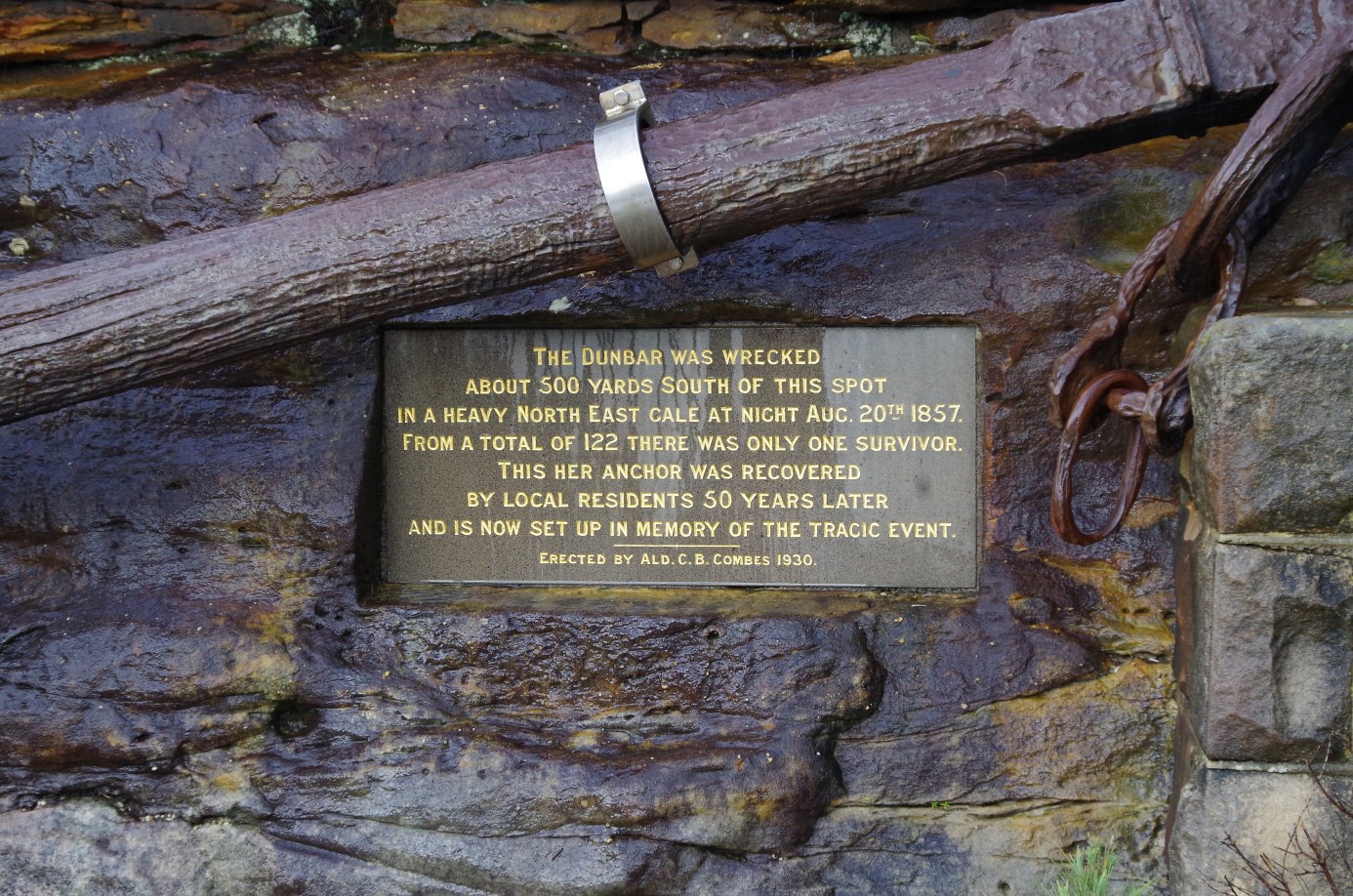This daytime outdoor photograph captures a detailed scene of a commemorative plaque embedded in a stone wall with hues of purple and gray. Centered on the rock wall, the dark gray plaque is notably reflective, possibly due to a glass covering, and is inscribed with yellow text. Above the plaque, a long wooden pillar secured with a silver metal clamp stretches diagonally from the lower left to the upper right. On the right side of the scene, three stone blocks are visibly stacked. The plaque reads: "The Dunbar was wrecked about 500 yards south of this spot in a heavy northeast gale at night, August 20, 1857. From a total of 122, there was only one survivor. This, her anchor, was recovered by local residents 50 years later and is now set up in memory of the tragic event. Erected by ALD.C.B.Combs, 1930."